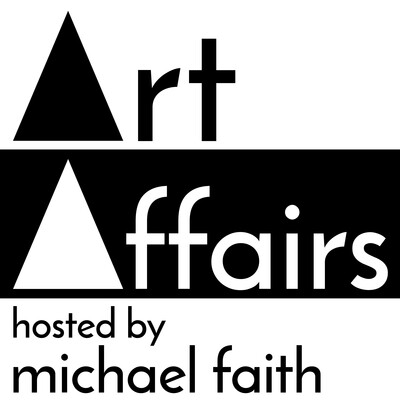The image displays a minimalist, black-and-white logo on a white background, advertising a media program titled "Art Affairs, hosted by Michael Faith." Dominating the design is the word "Art" in black text, with capital As represented by striking, filled-in black triangles. Below, the word "Affairs" is set in a black rectangular box, which features a white, hollow triangle as the capital A, followed by white text spelling out "F-F-A-I-R-S." Underneath, in a smaller, simple black font, it says "hosted by" on one line, and beneath that line, slightly larger text reads "Michael Faith." The text aligns to the left, contributing to the clean and straightforward aesthetic of the design.